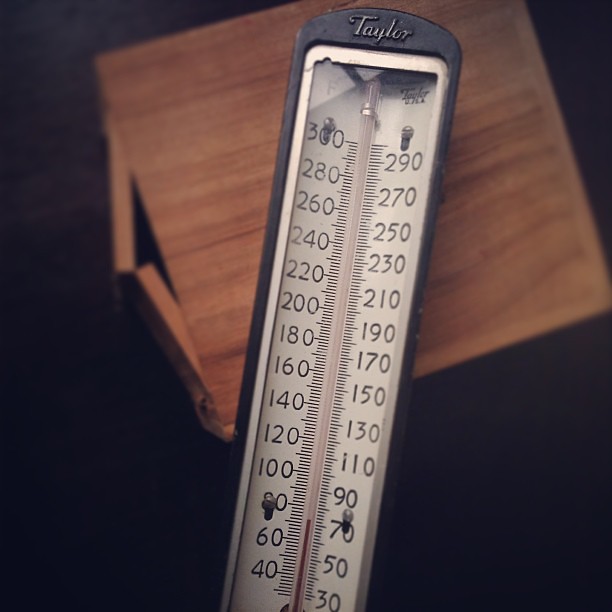A beautifully detailed image showcases a vintage wall-mounted thermometer. The thermometer is encased in an elegant wrought iron black metal frame, exuding a classic charm. At the top, the brand logo "Taylor" is prominently featured. The thermometer face is white, with clear, black numbers for easy readability. The temperature is indicated by a long glass tube filled with red liquid, which currently reads 72 degrees Fahrenheit (22 degrees Celsius). The Fahrenheit scale is on the right, while the Celsius scale is on the left, both accompanied by precise black lines for accurate measurement.

The thermometer is set against a backdrop of a rustic square wooden box with two doors, which are open on the left side, revealing its vintage character. This wooden box is positioned on what appears to be a sleek black fabric or countertop, adding a contrasting modern touch to the overall vintage aesthetic of the image.